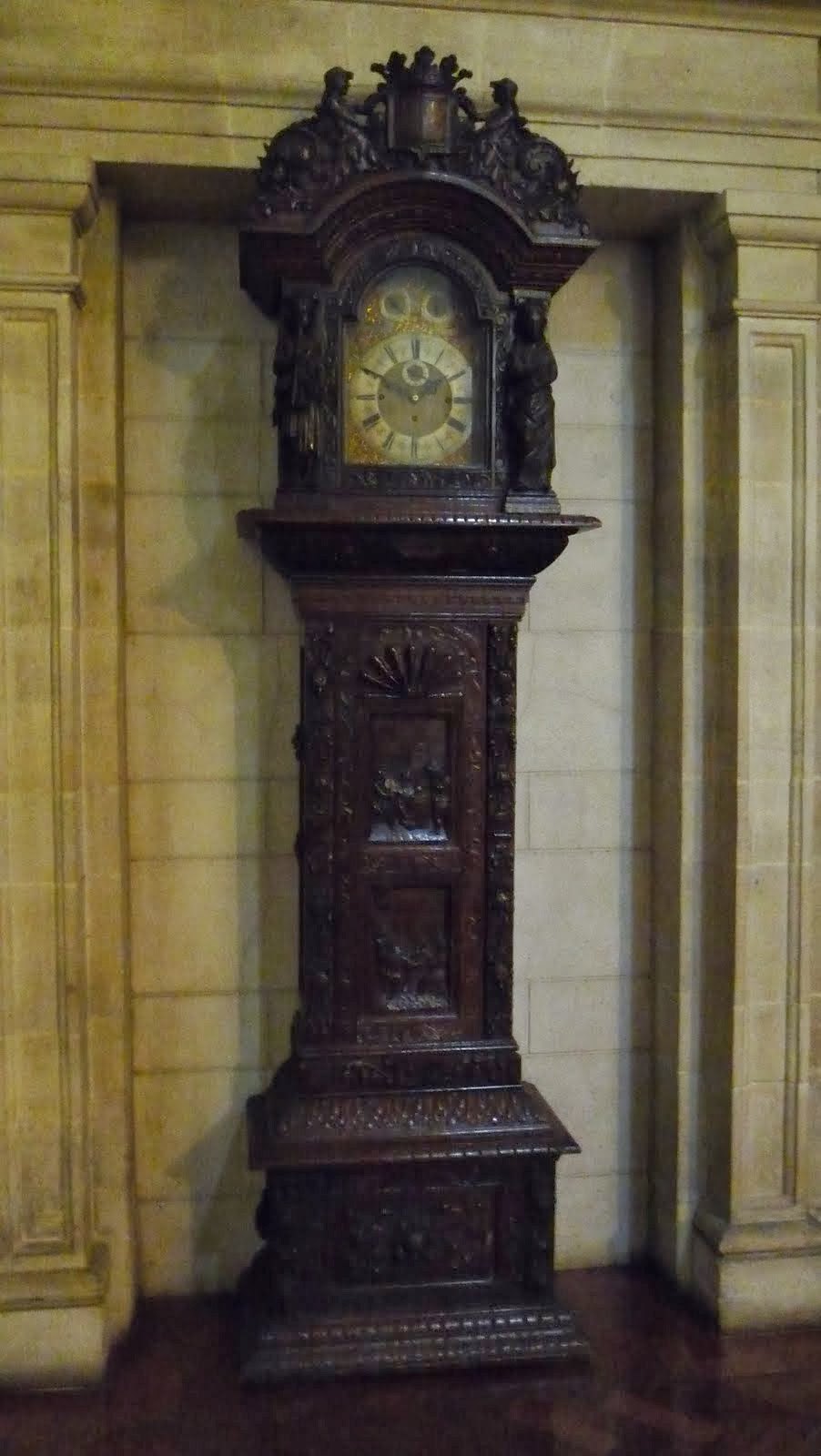This photograph depicts a majestic grandfather clock framed within a rectangular, portrait-oriented image. The clock, exuding an antique charm, features a dark, metallic, brownish-black exterior. Its ornate face, adorned in gold and white, displays bold black numerals. The clock is nestled in an alcove within an off-white wall, flanked by two elegant columns on either side. The floor beneath shares a similar dark brownish-black hue, harmoniously complementing the clock's stately appearance. The overall scene evokes a sense of timeless elegance and historical grandeur.